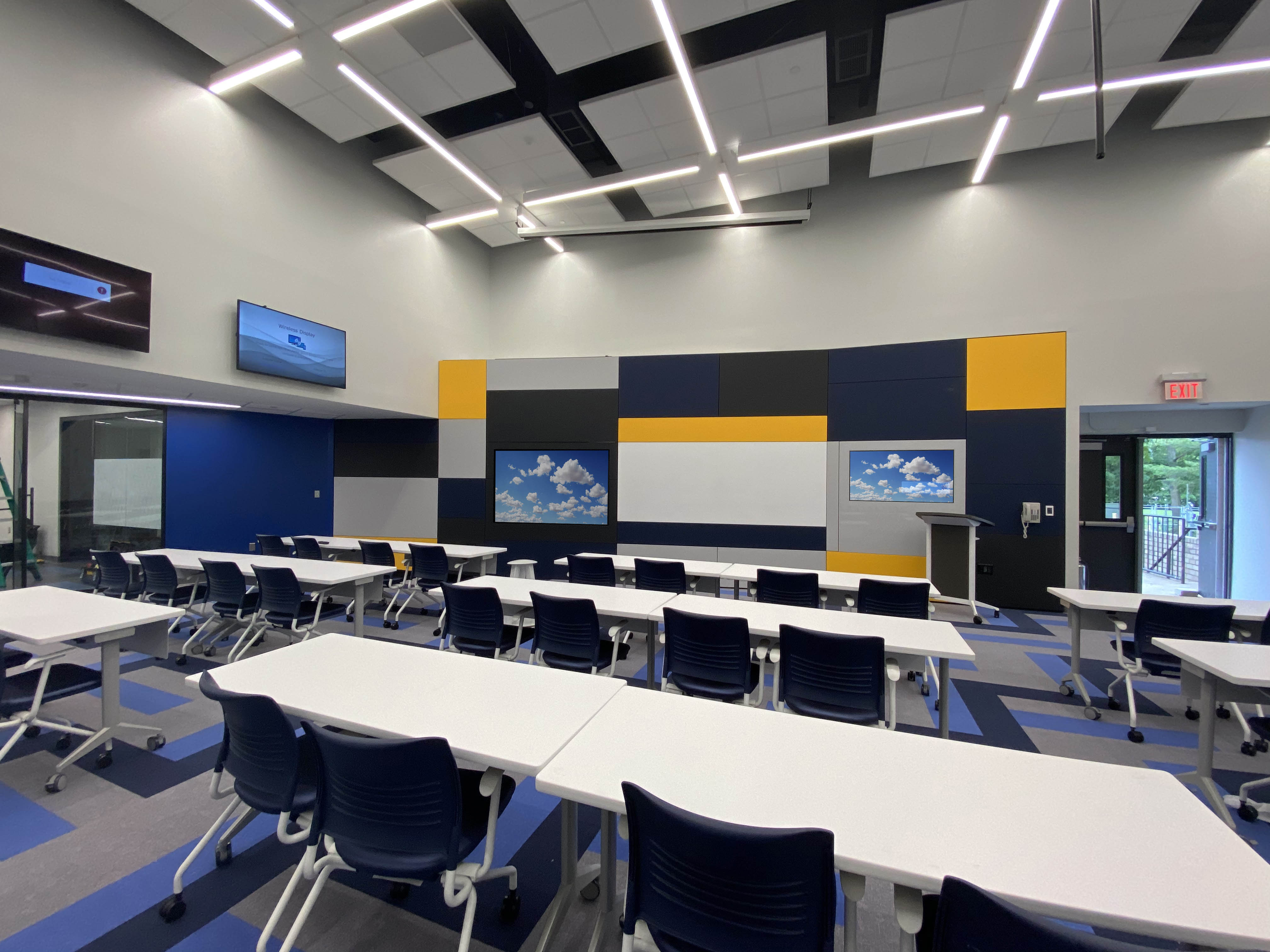This image captures an indoor space that appears to be a multifunctional room, likely used as a classroom or an office. The room features nine long, white rectangular tables arranged in rows, with each table accompanied by four blue chairs, some of which have wheels for easy mobility. The layout is designed to facilitate collaboration and interaction. In the front of the room, there appears to be an area designated for presentations, marked by a couple of screens. These screens are set against a backdrop adorned with dark blue, yellow, and gray square shapes, and feature images resembling a sky with clouds. 

To the left wall, additional screens are mounted overhead, while below, large windows provide a view into another part of the building, possibly revealing a staircase. The exit located on the far right has an open door with a red exit sign above it. A telephone is situated to the left of this exit. The room is illuminated by a series of ceiling lights, and the carpeting features a blend of blue, light blue, and gray hues, complementing the overall color scheme. The glass elements and open design suggest a modern, airy environment conducive to both learning and working.